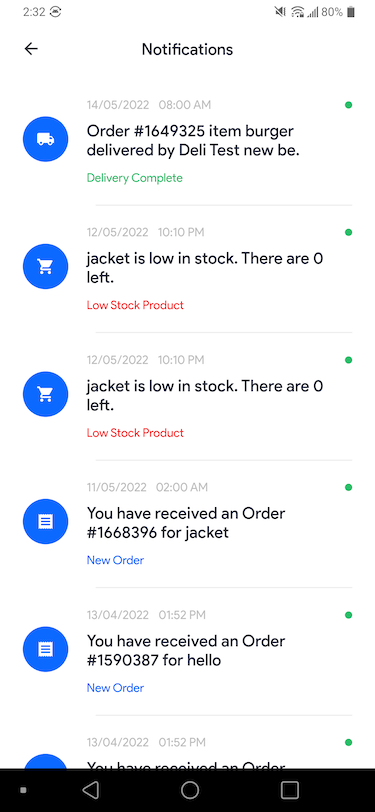A smartphone screenshot displays various notifications on a white background. The top status bar indicates the time is 2:32 and the battery is at 80%. There's a left-facing arrow at the top of the screen, with the word "Notifications" prominently centered below it. 

Beneath this, in gray text, the date "14/05/2022" is shown alongside the time "08:00 AM." The first notification features a blue circle with a delivery truck icon and reads: "Order number 1649325, item: Burger delivered by Deli Test New B." The status "Delivery complete" is highlighted in green.

Following this, another line indicates "12/05/2022 10:10 PM," with a blue circle containing a shopping cart icon. This notification states: "Jacket is low in stock, there are zero left," with the status "Low stock product" emphasized in red. Directly beneath, an identical notification repeats every detail.

Finally, listed under "11/05/2022 02:00 AM," another alert states: "You have received an order (number 1668396) for jacket."